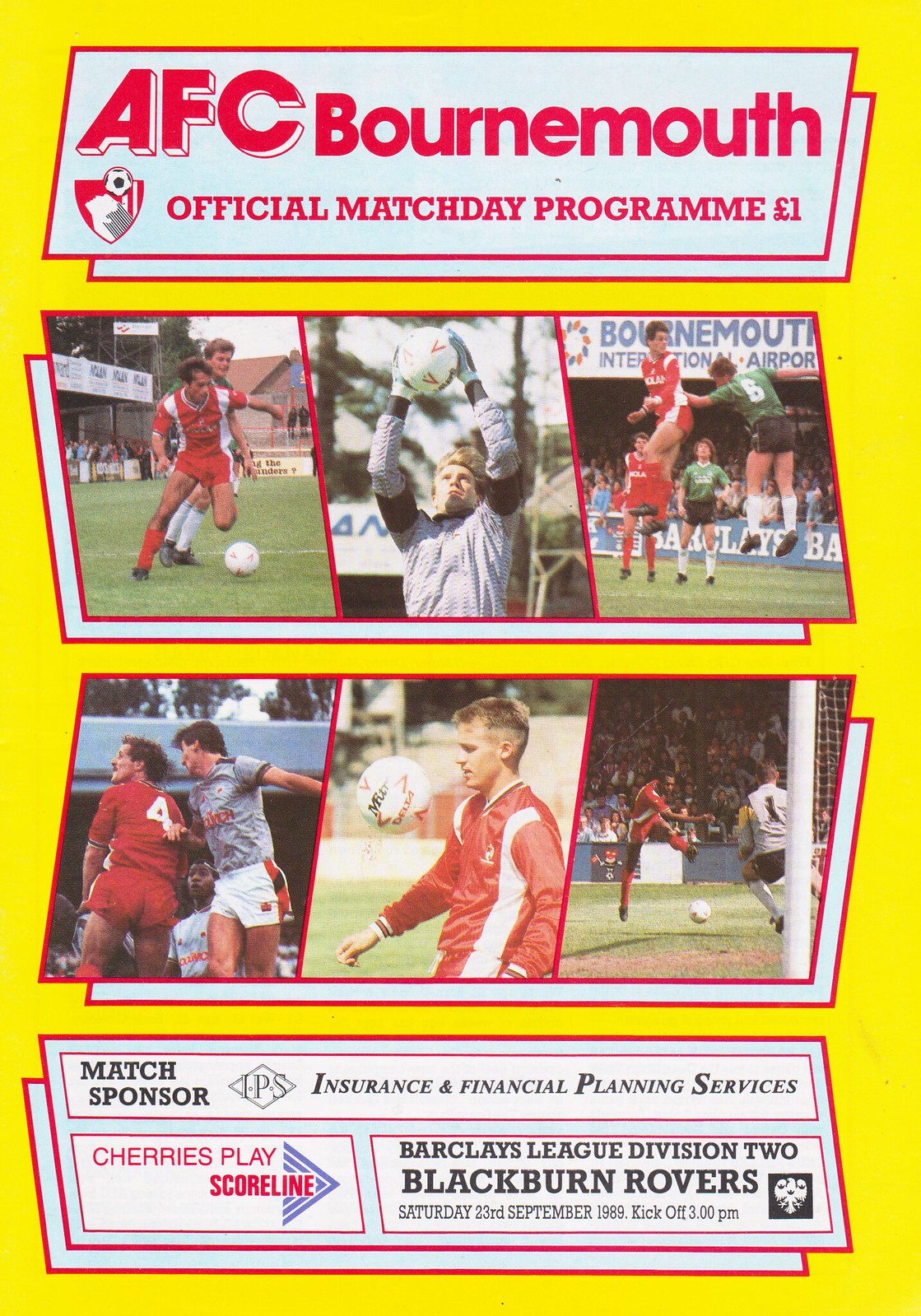The image is a color cover of a soccer program for AFC Bournemouth. The background is predominantly yellow with a red-bordered section at the top, where the title "AFC Bournemouth Official Match Day Program" is displayed, priced at one pound. To the left of this title is a small logo of AFC Bournemouth. Below the title section, there are two distinct rows of photographs, six in total, showing football players in various actions during a match. These photos are framed with white boxes and red outlines. Under these rows of photographs, there is another red-bordered area containing advertisements for IPS Insurance and Financial Planning Services. Additional texts on the cover include “Cherries Play Score Line” on the bottom left and details about the event on the bottom right, specifying "Barclays League Division 2, Blackburn Rovers, Saturday 23rd September 1989, Kickoff at 3 p.m."